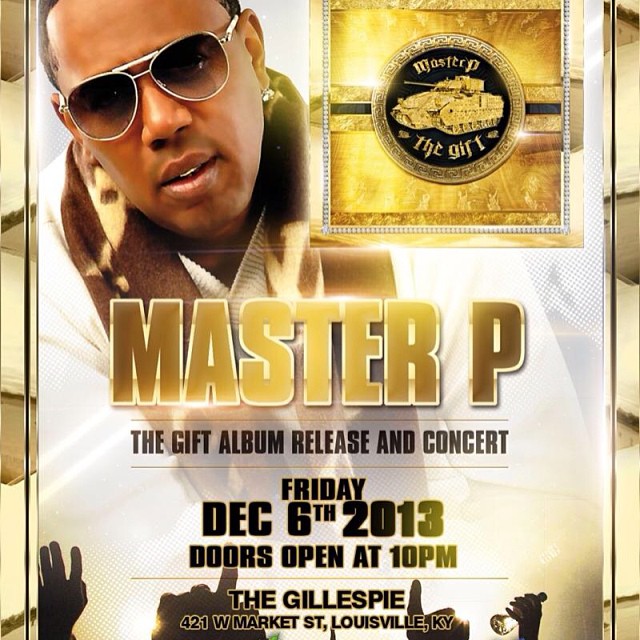This advertisement poster for Master P features a prominent headshot of the artist, a black man wearing sunglasses, an earring, and a white jacket with a gold collar over a white shirt. His mouth is slightly open, and he exudes an aura of confidence and style. To his right, there is a gold plaque with a decorative circle at the center, showcasing a golden tank and the text “Master P, The Gift,” surrounded by an opulent frame of gold, diamonds, and various jewels. Below this image, the poster announces in bold gold letters with a white outline, “Master P - The Gift Album Release and Concert.” The event details follow in black text, stating it will be held on Friday, December 6, 2013, with doors opening at 10 p.m. The venue is listed as The Gillespie, located at 421 West Market Street, Louisville, Kentucky. The bottom edge of the poster is adorned with darkened pictures of hands reaching up, possibly from a crowd, with one hand on the right side notably holding a microphone, adding to the concert atmosphere.